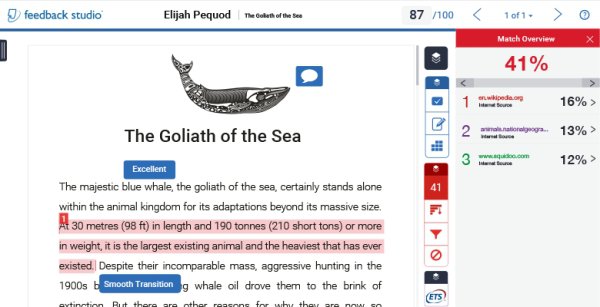The image showcases a screenshot from a learning application named "Feedback Studio," identifiable by its logo resembling a blue notepad with a cable in the top left corner. At the very top of the page, the document title, "Elijah Pequod, the Goliath of the Sea," is prominently displayed. The document in view is indicated as page 87 out of 100, marked as 1 of 1 in the pagination.

The central part of the screen features a white document displaying an illustration of a large gray whale, viewed from the side. A speech bubble from the whale contains the text: "The Goliath of the Sea." Beneath the illustration, a paragraph begins with a descriptive caption about the blue whale, emphasizing its status as the largest and heaviest animal ever recorded. The text highlights its impressive dimensions—30 meters (98 feet) in length and up to 190 tons (210 short tons). It also references the historical threat of aggressive hunting for whale oil in the 1900s, noting the brink of extinction faced by the species. The provided text cuts off mid-sentence.

The document also includes various annotations: a blue button labeled "Excellent" and another labeled "Smooth Transition," with certain sections of text highlighted in pink for emphasis or correction. On the right-hand side of the screen, a "Match Overview" displays a similarity index of 41%, with one of the primary sources noted as "wikipedia.org." This sidebar suggests the text's originality is being checked against existing online sources.